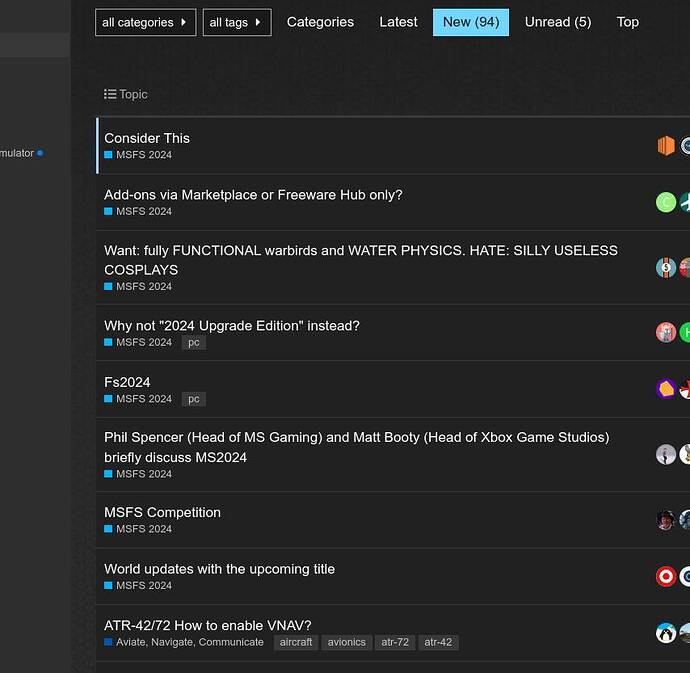In the image, a dark-themed screen showcases various categories and tags related to content—highlighting sections such as 'Categories', 'Latest', 'New', and 'Unread.' The 'New' section indicates there are 94 new items, with 5 unread items specifically tagged under 'Top'. The display also features a blue "MSF 2024" label next to all categories. 

Additionally, there's a message prompting users to consider add-ons via the Marketplace or Freeware Hub, querying preferences for functional war birds and water physics, while expressing disdain for frivolous cosplays. It suggests upgrading to a 2024 edition and mentions "FS 2024," in the context of Phil Spencer and Matt Booty briefly discussing competition, world updates, and enabling VNA for an upcoming title. The layout and text orientation hint at an interface related to email or a content management system, yet it lacks sufficient detail to definitively identify its purpose.